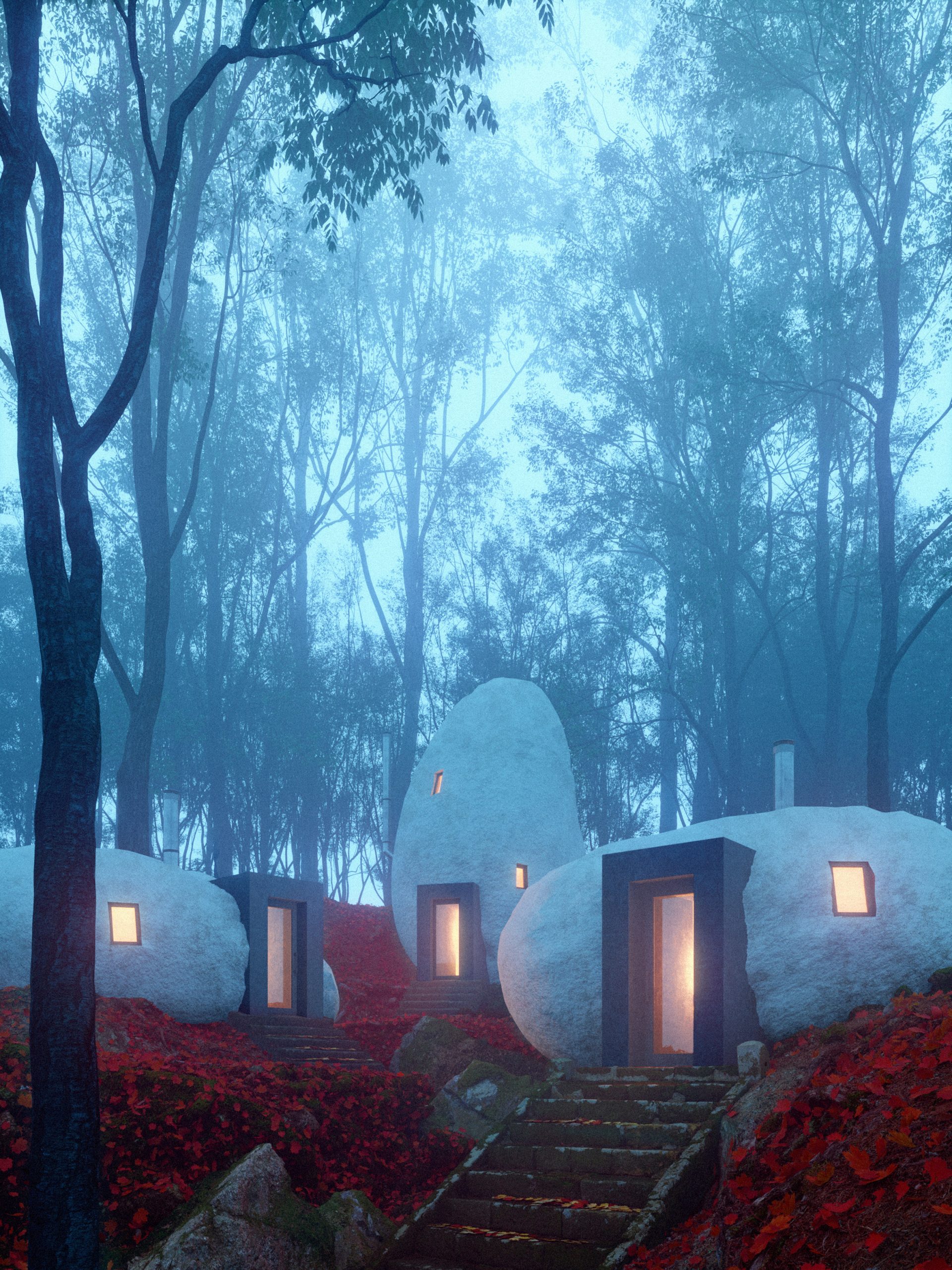In a vertically-oriented, realistic but somewhat blurry and painterly image, three curious white structures dominate an outdoor scene. Resembling small, round river rocks or igloos sans the snow, these three elliptically shaped buildings exude an almost ethereal glow, with warm light streaming from their thick, dark-bordered doorways and small windows. Crafted seemingly from materials like adobe or a smooth, resilient paper mache, each orb-like building features a rustic, brown staircase leading up to its inviting but mysterious entrance. Smokestacks hint at their functionality, suggesting a permanence beyond a movie set facade. The background is a foggy, pale blue sky interwoven with the stark black trunks of tall, slender trees, whose sparse leaves add to the eerie, sci-fi ambiance. Surrounding the bases of these white orbs are vibrant, textured red flowers that seem to thrive in this otherworldly environment, adding a contrasting burst of life to the strange architectural tableau.